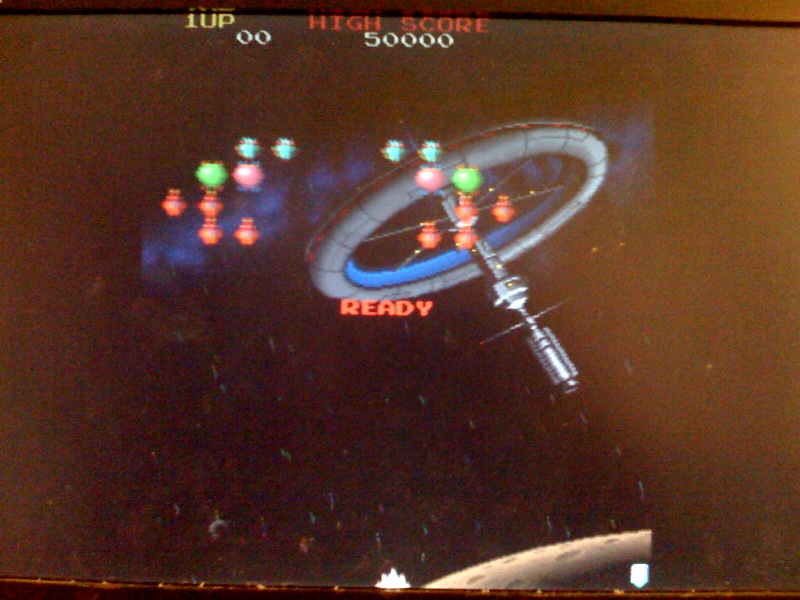The screenshot captures a scene from what appears to be a retro-style computer game. The background features a gradient of brown hues, darker on the left side and transitioning to lighter shades on the right. Centered in the image is a spaceship, characterized by a large gray circular main body with a protrusion extending diagonally downward toward the lower right. This protrusion is rendered in a silver tone.

Adjacent to the spaceship is a collection of colorful elements suggesting a HUD or some form of game interface. This includes a small section of blue gas and an array of circles in various colors: four red, one light green, one pink, and two white. The spaceship itself mirrors these colors with two white circles, one pink, one light green, and four red circles situated on or near the vessel.

At the bottom of the spaceship, the word "READY" is prominently displayed, indicating the player's readiness status. The top of the screen features "1 UP" and "HIGH SCORE" labels, with "1 UP" showing a score of 0000 and "HIGH SCORE" displaying a score of 50,000.

Additionally, there are subtle gray lines depicted below the spaceship, possibly representing thrusters or movement. The lower section of the screen shows a small portion of a brown planet or moon, adding to the scene’s outer space ambiance.